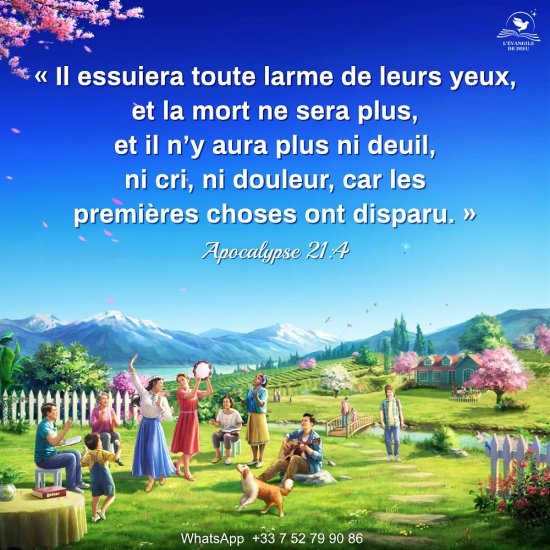The illustration depicts a vibrant outdoor scene with a family and friends joyfully playing music, dancing, and picnicking on a lush green lawn. To the left, a white picket fence frames the area, and a wooden bridge spans a small river at the back of the lawn. Across the river lies a charming blue house with a red roof, surrounded by trees adorned with pink cherry blossoms. In the distance, majestic green and snow-capped blue mountains rise against a brilliant blue sky. A yellow-tableclothed table with a red book rests in the bottom left corner. White text in the center-bottom reads "WhatsApp +33 7 52 79 90 86," indicating contact information. White French text, appearing to be a Bible quote or notable saying, is emblazoned at the top against the sky, complemented by a logo of a dove and book in the top right corner. The intricate details and lively atmosphere capture a moment of joyous outdoor celebration and natural beauty.